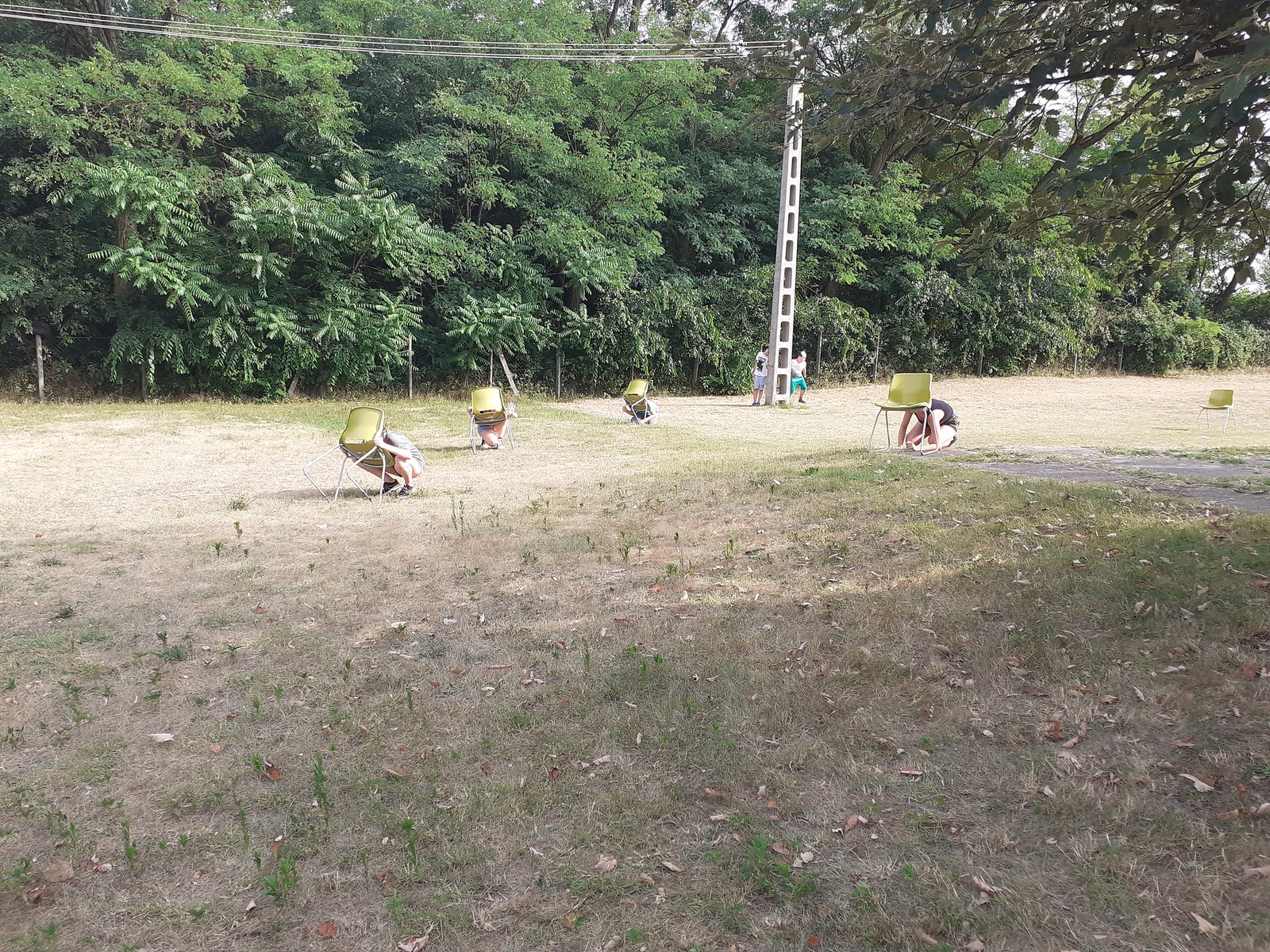The photograph captures a peculiar scene set in a slightly unkempt field of brown and green grass, bordered by a thick tree line. In the middle of the field, there are five lime green bucket chairs with metal legs scattered at various distances from each other. Four people, three of whom appear to be women and one possibly a man, are squatting or kneeling behind these chairs, using them to cover their heads. Each person is separated by a few feet, hiding or ducking in different positions, with one chair left empty among them. 

On the right side of the image, a person dressed in a black tank top is seen kneeling on the ground, their head also hidden beneath a chair. Across from them, another individual in a gray shirt is grabbing a chair, seemingly about to put it over their head. 

Towards the far end of the field, there is a gray cinder block tower, possibly a power utility pole, with telephone lines stretching across. Next to this tower, a man and a woman are standing side by side; the man appears to be preparing to run. Additionally, there is a small patch of concrete visible in the field, adding to the scene's odd yet intriguing ambiance. Leaves from overhanging trees partially frame the photograph, enhancing the natural but peculiar setting.